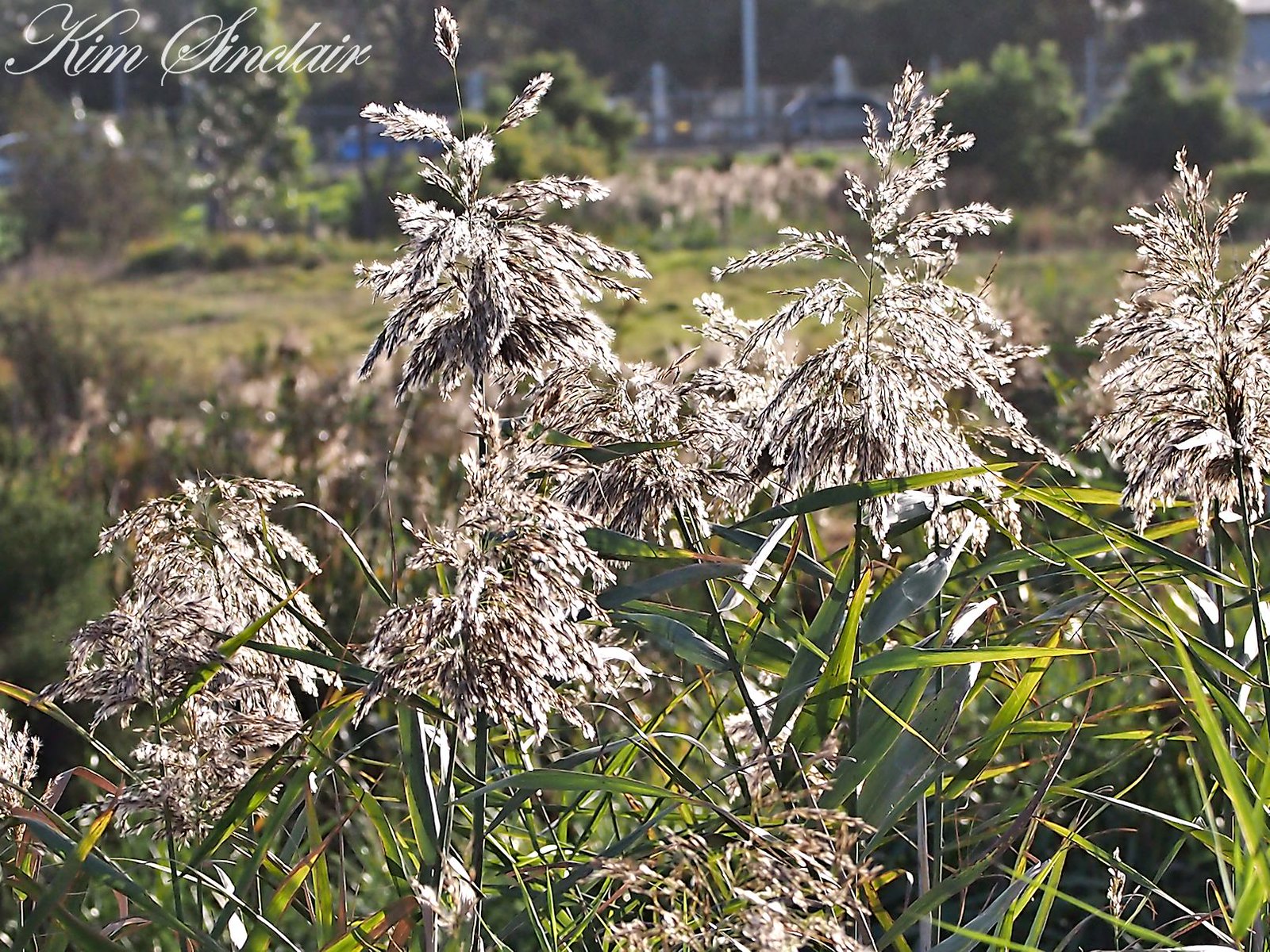In this photograph, a cluster of off-white, wheat-like plants is seen sprouting from the ground, interspersed with green leaves. The detailed close-up captures the intricate textures and natural beauty of the plants. In the background, slightly out of focus, a blurry field stretches out, with what appears to be a farmhouse faintly visible on the distant horizon. The top left corner of the image features the name "Kim Sinclair" inscribed in white text. The overall composition beautifully blends the foreground's botanical details with the serene, pastoral backdrop.